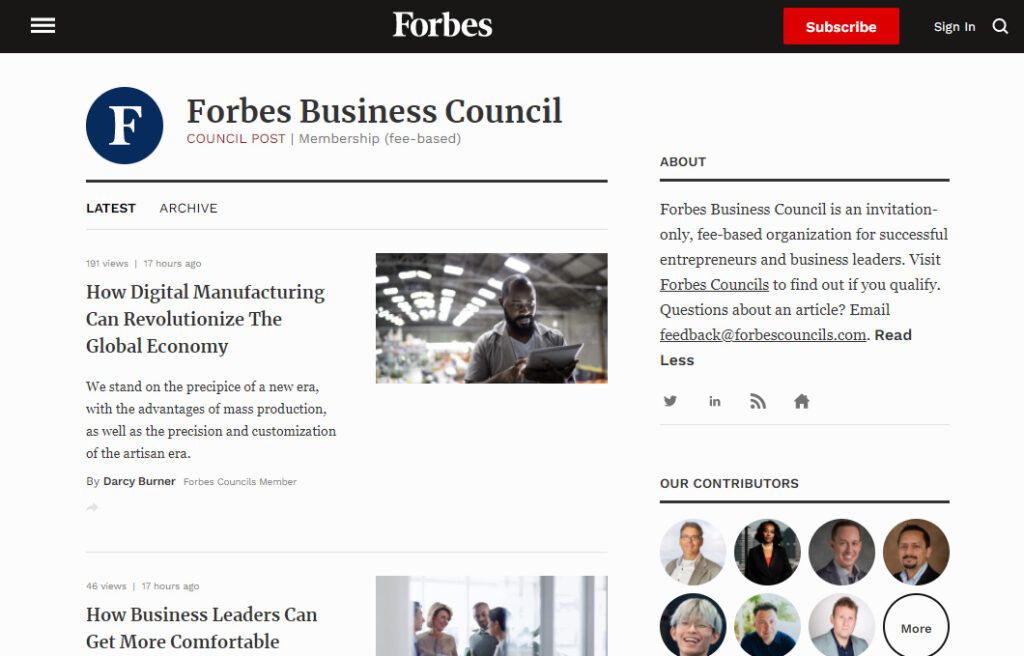The image features a detailed infographic for the Forbes Business Council, encapsulated within a visually appealing design. At the top, the image includes a series of line marks and dash marks which blend into an illustration of a hammer, indicating the idea of construction and effort. To the left, a bold "Forbes" logo is prominently displayed.

A red rectangle located next to the hammer illustration contains the text, “The Sky is the Limit,” alongside a magnifying glass icon that symbolizes scrutiny and in-depth analysis. The color scheme of the infographic features vibrant hues of red and blue, centering around a large "F" that represents Forbes.

The title "Forbes Business Council" and "Council Post" are distinctly highlighted, with subsections detailing "Membership," "Feedbase," "Latest Archive," "1A1 View," "Centennial High School," "Digital Manufacturing," "Conversion," and "Global Economy."

The infographic underscores a thought-provoking article by Darcy Brenner, a member of the Forbes Council. The article delves into the changing landscape of business, emphasizing how leaders can adapt to new eras of invention, mass production, and personalized customizations within the arts.

Below, there is text informing readers about the exclusive nature of Forbes Business Councils, describing it as an invitation-only organization dedicated to successful entrepreneurs and business leaders. A call-to-action invites curious readers to visit the Forbes Councils’ website to determine if they qualify for membership.

For readers who have questions about the article, a point of contact is provided: feedback@ForbesCouncils.com.

At the bottom, icons for social media such as Twitter, LinkedIn, and a "Holify" option are depicted, encouraging contributions and further engagement. The closing note mentions that additional text on Forbes News for Contributors is available. 

The infographic brings together a blend of professional insights, exclusive invitations, and calls to action, making it a comprehensive guide for Forbes Business Council members and potential applicants.